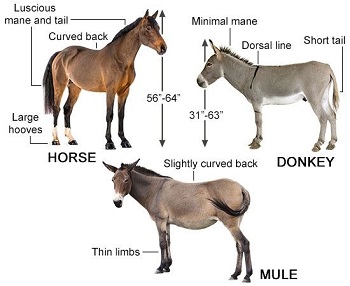The image features a detailed educational chart against a white background, illustrating and comparing three different animals: a horse, a donkey, and a mule. Each animal is adorned with descriptive labels connected by dark arrows explaining their distinct features. 

The horse, positioned on the upper left, is brown with black and white accents. Labels highlight its luscious mane and tail, curved back, and large hooves, specifying its height range from 56 to 64 inches from ear tip to the ground. 

To the horse's right is the gray donkey, which has a white belly and black accents. Its labels note a minimal mane, a dorsal line, a short tail, and a height ranging from 31 to 63 inches. 

The mule, located in the lower half of the image, displays a mix of black, white, gray, and lots of brown. It has thin limbs, a slightly curved back, a black nose with a white snout, and long ears.

The chart aims to educate viewers on the differences between these often-confused animals, emphasizing their unique physical characteristics with all descriptive text in black and neutral colors used for the animal depictions.